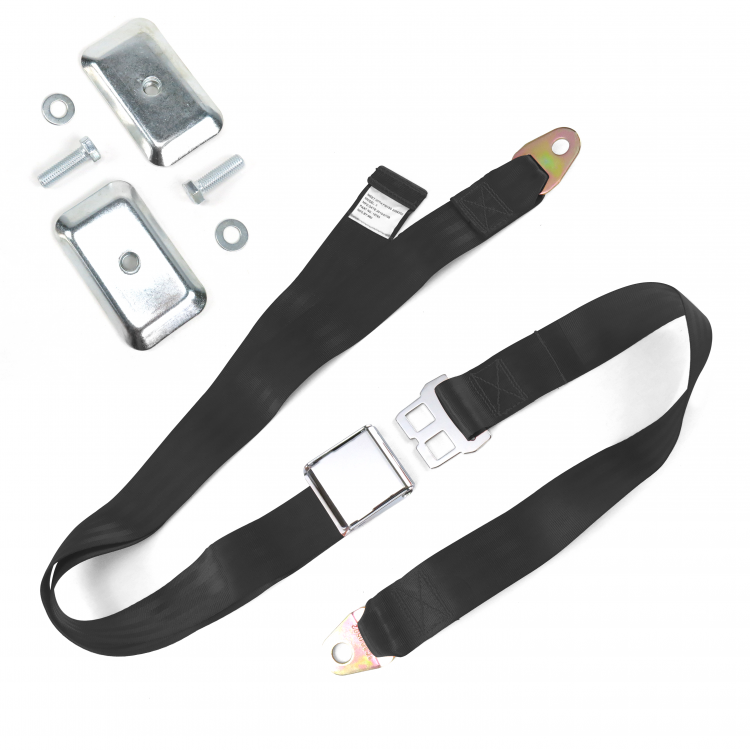This detailed photo depicts a black woven seatbelt lying on a pristine white background. The seatbelt, featuring silver hardware, resembles the kind typically found in airplanes, with a top-lifting mechanism to release the lock. At either end of the seatbelt are triangular metal pieces with holes, indicating where screws would attach it to a seat. Positioned around the seatbelt is an array of hardware: two metal rectangles with drilled holes, two screws, two nuts, and two washers, all meticulously arranged. The seatbelt itself is displayed with an S-shaped curve, accentuating its sleek double-layered material. The overall arrangement showcases the belt and its corresponding parts, suggesting an assembly process.